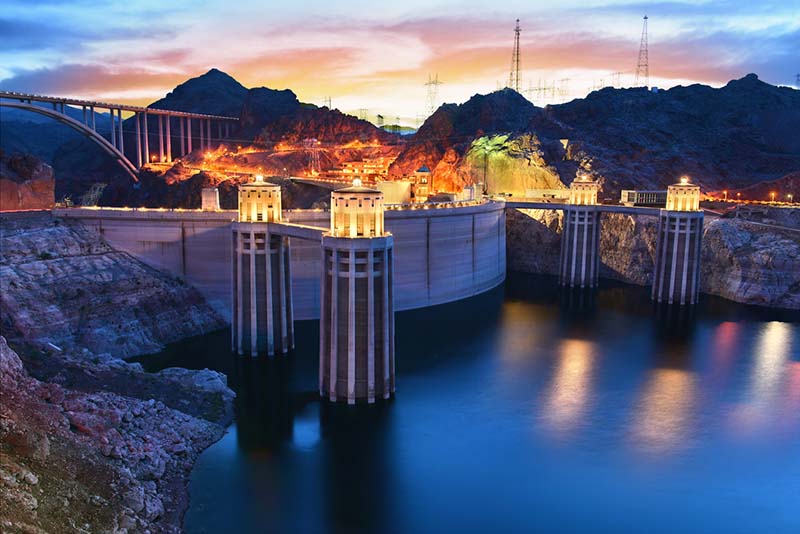As the sun sets, painting the sky in breathtaking hues of blues, whites, reds, oranges, and pinks, the image captures an outdoor scene dominated by a majestic mountain range. Below the dramatic tapestry of clouds that blanket the heavens, a curved dam is prominently featured, holding back a still body of water that stretches into the foreground. The dam is flanked by four brightly lit towers, and construction activity can be seen near a small valley in the mountains. On the left side of the scene, a large arched bridge begins its span across the valley, disappearing behind the mountainous terrain. Rock formations frame the waterway, topped by a roadway with lights beginning to flicker on, hinting at evening's arrival. In the distance, roads winding up to a quaint town can be seen, casting a warm glow against the encroaching twilight.